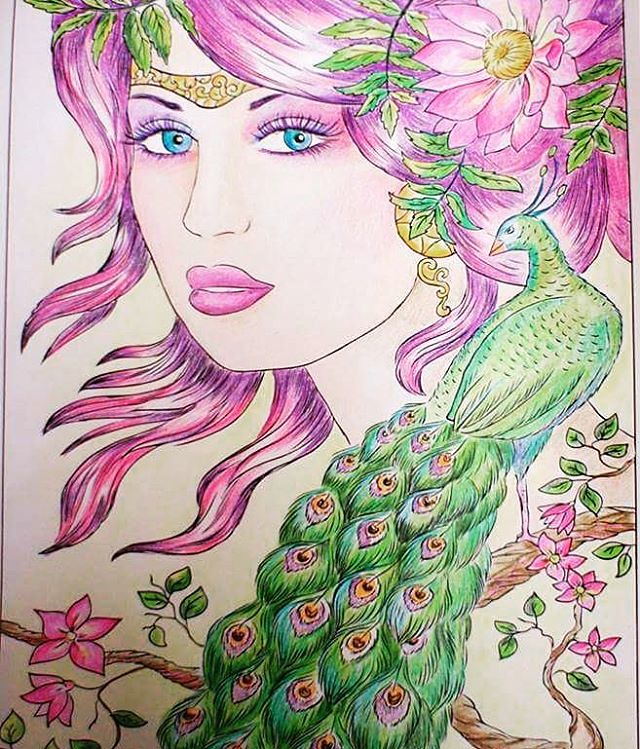The image is a detailed and vibrant portrait-style drawing on a white coloring book page. At the center of the composition is a goddess-like woman with radiant blue eyes. Her long, wavy pink hair cascades around her face, adorned with a pink flower on her left side, partially covering her ear, and strung with leaves. Gold circular earrings dangle from her ears, and a delicate, gold-like crown with leaf motifs rests on her forehead. Her complexion appears natural with pink puckered lips. Sharing the scene with the woman, a greenish-blue peacock with a long, eye-patterned tail stands regally on a brown tree branch that extends from the right side of the image. The branch is decorated with small pink flowers and green leaves, enhancing the intricate and colorful nature of the artwork.